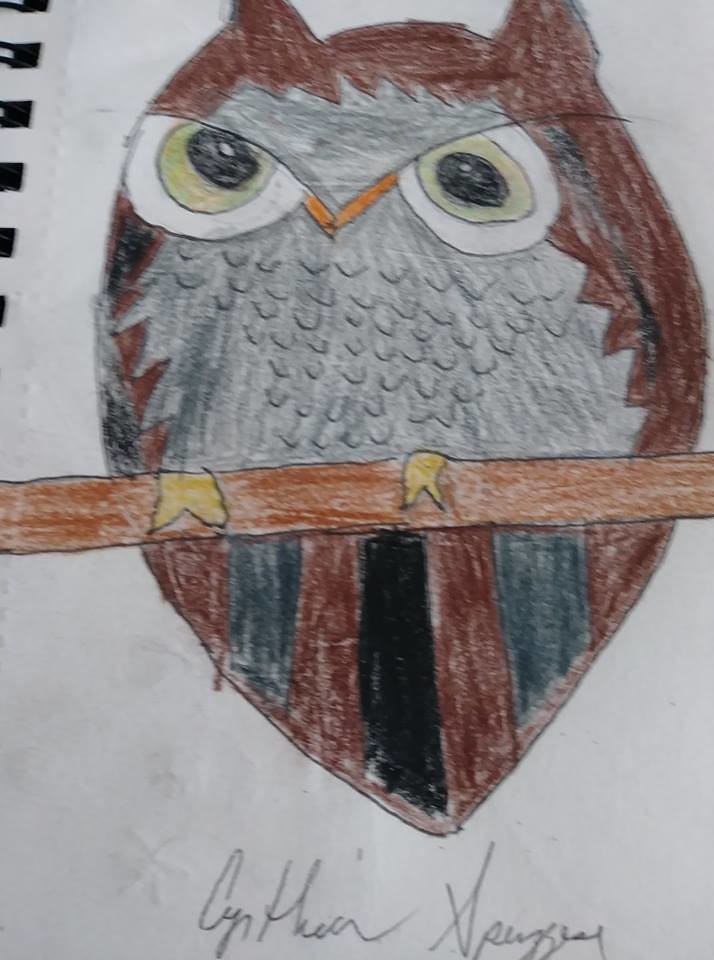This image is a detailed crayon drawing on a plain white sheet of paper torn from a spiral notebook, evident from the spirals in the upper left corner. The drawing portrays a prominently featured owl with a bulbous body perched on a horizontal brown branch that stretches across the middle of the picture. The owl displays a blend of brown feathers on its back and gray on its fluffy chest, enhancing its childlike yet expressive appearance. It has strikingly large green eyes and a small, orange beak. The owl's tail feathers exhibit gray and black stripes, and its yellow feet are clinging to the branch in a somewhat two-dimensional, almost pasted-on manner. Beneath the owl, there is a handwritten signature in pencil that reads "Cynthia," though the last name remains partly illegible. The careful outlines and coloring suggest both rudimentary and intentional detail, capturing the charming innocence of a child's artwork.